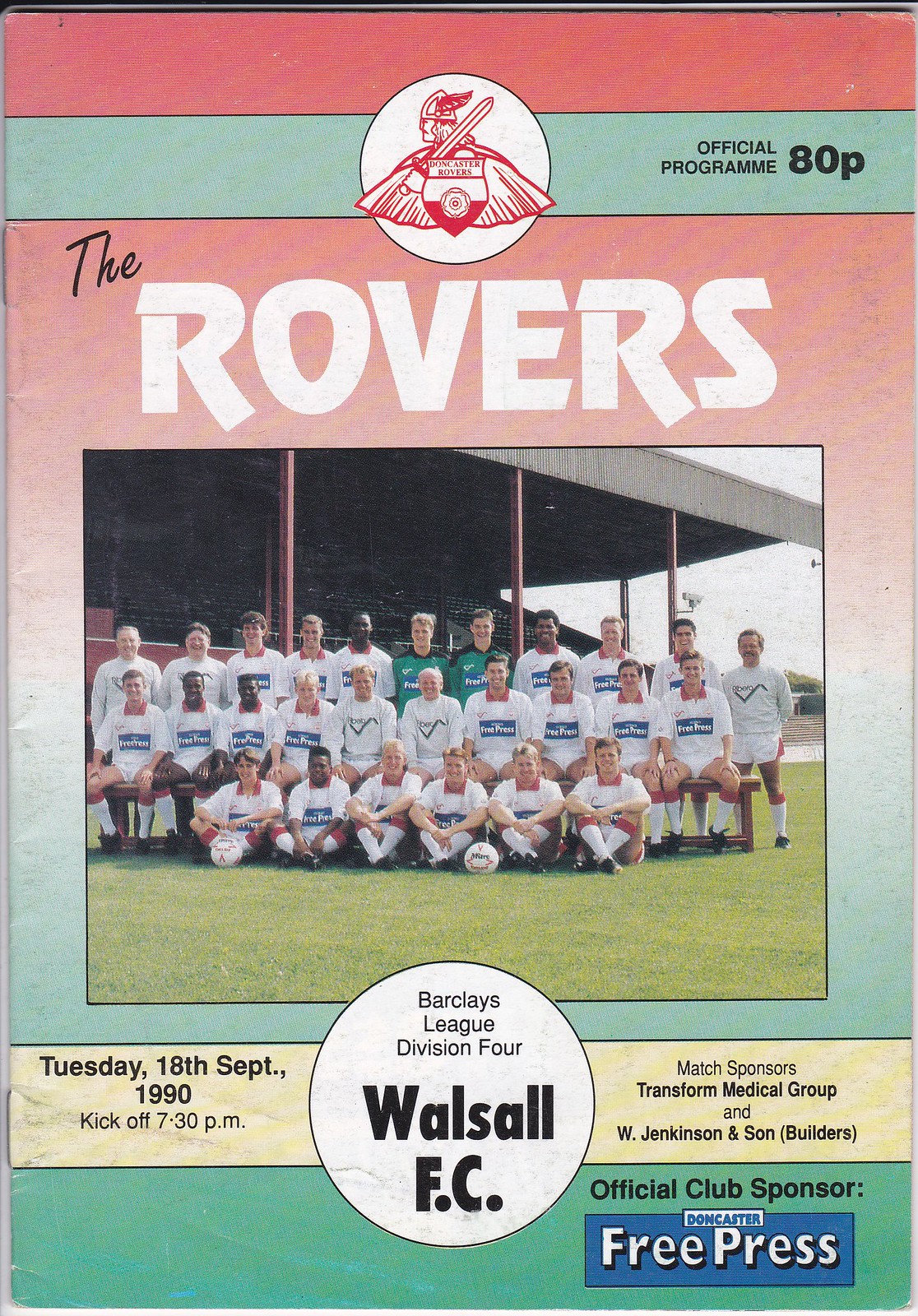The cover of the soccer program is a vertically aligned rectangular image featuring a gradient design with a red top, a white middle section, and a green bottom. Dominating the top section is the name “ROVERS” in bold white letters, accompanied by the emblem of the team, which depicts a Spartan-like figure with a helmet and sword, standing in front of a shield emblazoned with "Doncaster Rovers." Below the title, a group photograph captures the soccer team lined up in three rows on the grassy field of their stadium. Most players are dressed in white jerseys with a blue banner across the middle, while two players, presumably the goalkeepers, are in green jerseys. The team's white shorts and white socks with red stripes contrast against the green field and the stands visible behind them under a partly cloudy sky.

In the middle, there's a prominent section with a white circle that states, "Barclays League Division 4 Walsall FC" in bold black print, with "Walsall FC" specifically highlighted. To the left of the circle, it reads, "Tuesday, 18 September 1990," and mentions the kickoff time as 7:30 p.m. To the right, it lists the match sponsors as "Transform Medical Group and W. Jenkins and Sons (Builders)." The bottom left of the cover features another green bar, repeating the match date and time, while the bottom right corner states, "Official Club Sponsor: Doncaster Free Press." The price of the official program is noted as 80 pence in the bottom section.